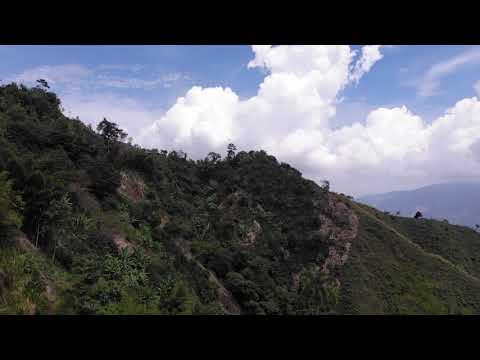The image depicts a scenic hillside adorned with green grass, bushes, and clusters of trees. A black border frames the top and bottom of the picture. The sky above is a vibrant blue, dominated by a large, puffy white cloud at the center-right. The foreground shows trails weaving through the green terrain, leading the eye towards the hilltop. In the background, another hill with a blue hue suggests a distant, similarly verdant landscape. The overall composition captures the serene beauty of nature with a clear, crisp sky and lush, green foliage.